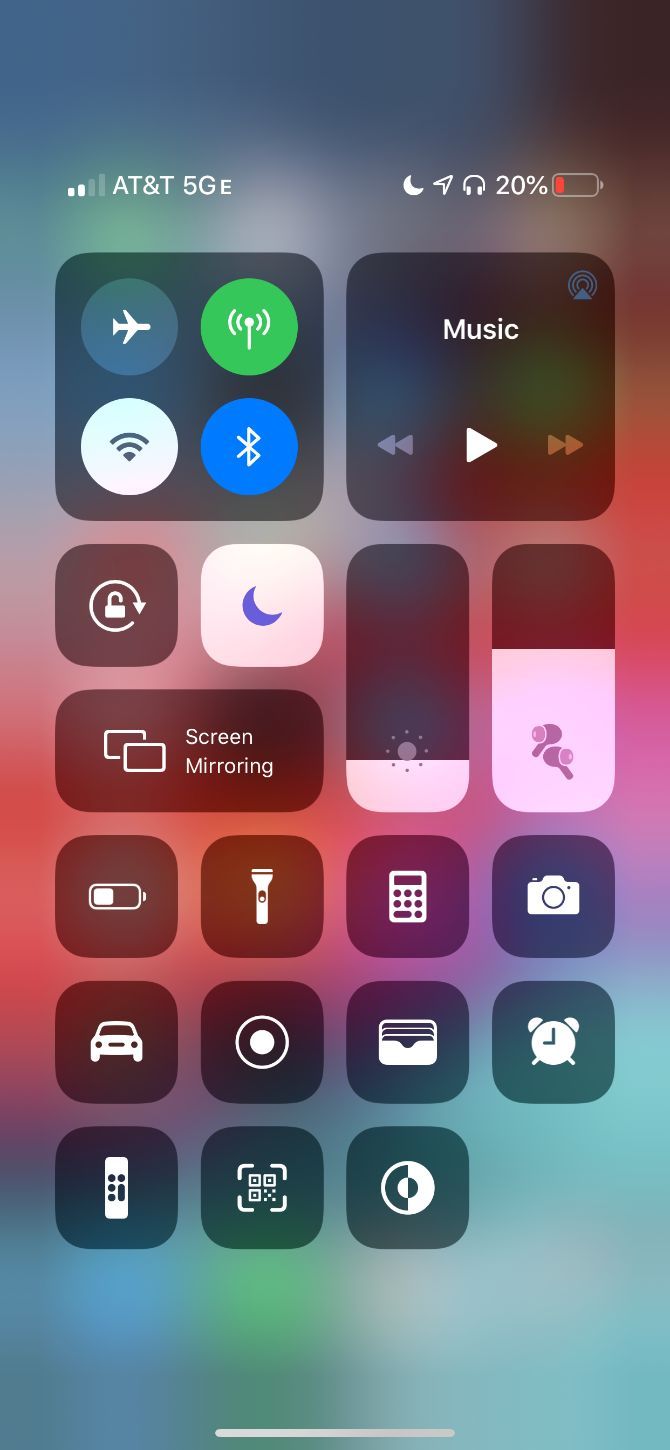This image is a screenshot of a phone's control center. The background is a gradient of vibrant colors transitioning from blue at the top to green at the bottom, but it's somewhat blurry. 

At the very top left corner, the phone signal strength is shown with four white bars, but only the first two bars are lit up. Next to this, "AT&T" is displayed, followed by "5G" and a small "E". On the right side, there's a small white crescent moon icon, an upwards-and-rightwards pointing arrow, a headphone icon, the text "20%" indicating battery percentage, and a battery icon showing a red line at the bottom, suggesting low battery.

Below this status bar, there are two black boxes side by side. The left box contains four circular icons: 
1. A blue circle with a white airplane.
2. A green circle with a white stick figure with two signal lines on top, indicating cellular data.
3. A white circle with a Wi-Fi symbol.
4. A blue circle with the Bluetooth logo.

The right box is labeled "Music" in white text at the center, with a small blue circle in the upper left corner. Below this are play controls: two left-pointing arrows for rewind, a play arrow, and two right-pointing arrows for fast forward.

Under the left black box, there's another black box with a white lock icon encircled by a nearly closed white line with an arrow pointing at the gap. Next to it is a white box with a blue moon icon.

Below these, there's a longer rectangular black box labeled "Screen Mirroring" with two overlapping white squares on the left. Next to this is a vertical black rectangle with a white bottom featuring a central gray circle surrounded by three smaller gray dots.

Following this, there's a vertical rectangle transitioning from black to red and then to white with a purple-mauve logo inside, though the logo is indistinct.

Further down, there are multiple black boxes with various white icons inside: 
1. A battery icon.
2. A flashlight symbol.
3. A calculator.
4. A camera icon.
5. A car icon.
6. A white circle surrounded by a thin white outline circle.
7. A wallet icon with three lines indicating the presence of credit cards.
8. An alarm clock.
9. A remote control-like icon.
10. A box made up of four corner lines with a smaller box inside composed of four smaller boxes.

Each icon and element is thoughtfully positioned to provide quick access to essential functionalities and information.